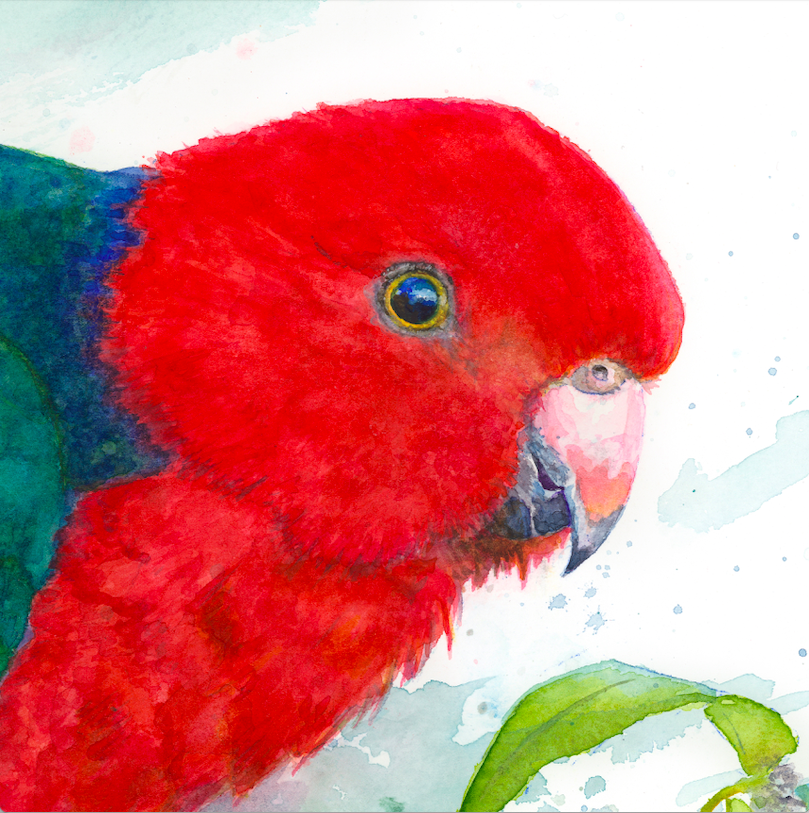This artwork is a detailed watercolor drawing of a parrot, prominently featuring its head and upper chest, which are covered in vibrant red feathers. The bird's plumage transitions from red to blue and then green as it moves towards the back, although only a small portion of its body is visible. The parrot has a distinctive beak that is shaded in gray, pink, and white, with a sharp edge. The eye is striking, with a black center surrounded by yellow, and an outer ring of darker brown. In the lower right-hand corner of the composition, a green leaf adds a touch of realism and balance to the image. The background is predominantly white with light blue watercolor washes, creating a serene and airy atmosphere.